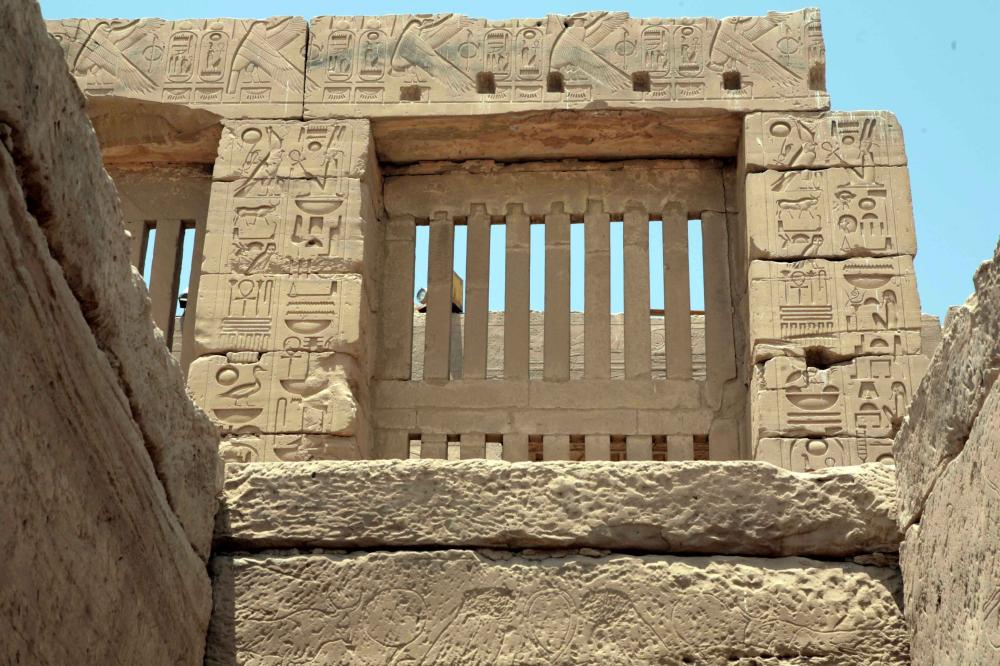This photograph captures an upward view of an ancient Egyptian ruin from below. At the bottom of the frame, light beige stone slabs form the base, extending upwards into both the left and right sides. Dominating the center of the image are two imposing stone pillars, intricately carved with hieroglyphs depicting various animals, people, figures, dishes, and other objects. These hieroglyphs, though weathered, add a layer of historical depth and character to the scene. Between the pillars, a formidable gate resembles a jail cell, formed from horizontal and vertical stone slabs. Above the gate is a large right-angled stone cap, also adorned with hieroglyphs. To the left, another similar setup is partially visible, hinting at a larger architectural complex. The backdrop of the image includes a pale blue, almost yellowish sky, adding a serene contrast to the ancient stonework. The ancient and intricate carvings on every surface offer a glimpse into the sophisticated artistry of ancient Egypt, despite the weathered state suggesting centuries of exposure.